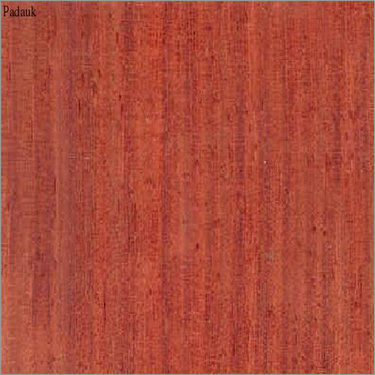The image showcases a close-up view of a square-shaped wooden plank, possibly resembling a tile or piece of flooring. The wood exhibits a rich reddish-brown hue, reminiscent of cherry or mahogany, with prominent darker and lighter streaks running vertically, delineating the grain. These grain lines, coupled with the wood's natural striations, suggest an intricate texture with lighter brown bare spots scattered throughout. The plank is somewhat shinier in the middle compared to the edges. In the upper left-hand corner of the plank, there is black text, with the word "PADAUK"—the 'P' is capitalized, and the rest of the letters are in lowercase. The detailed grain and speckled appearance enhance the textured aesthetics of the wood.